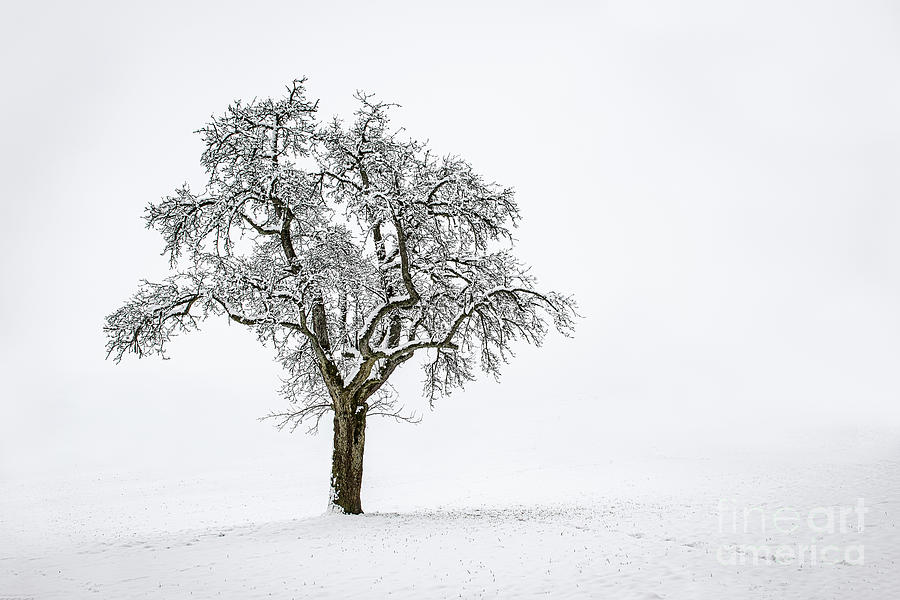This striking image, likely a photograph with a Fine Art America watermark in the lower right-hand corner, captures a solitary tree in a stark, snowy landscape. The tree, positioned slightly left of center, is the main focus, standing tall with intricate, sprawling branches devoid of leaves and dusted with snow. The background is an unbroken expanse of white, suggesting a seamless transition between the snow-covered ground and the overcast sky, adding to the sense of isolation. A subtle gradient of grays creeps in from the edges, enhancing the minimalistic and stark atmosphere. There are delicate details of grass poking through the snow near the base of the tree, and a faint silhouette of mountains can be discerned in the distant background on the right side, emphasizing the depth and vastness of the wintry scene. The overall tones of the image are predominantly white and black with a hint of pale brown on the tree, enhancing its starkness against the snowy backdrop.